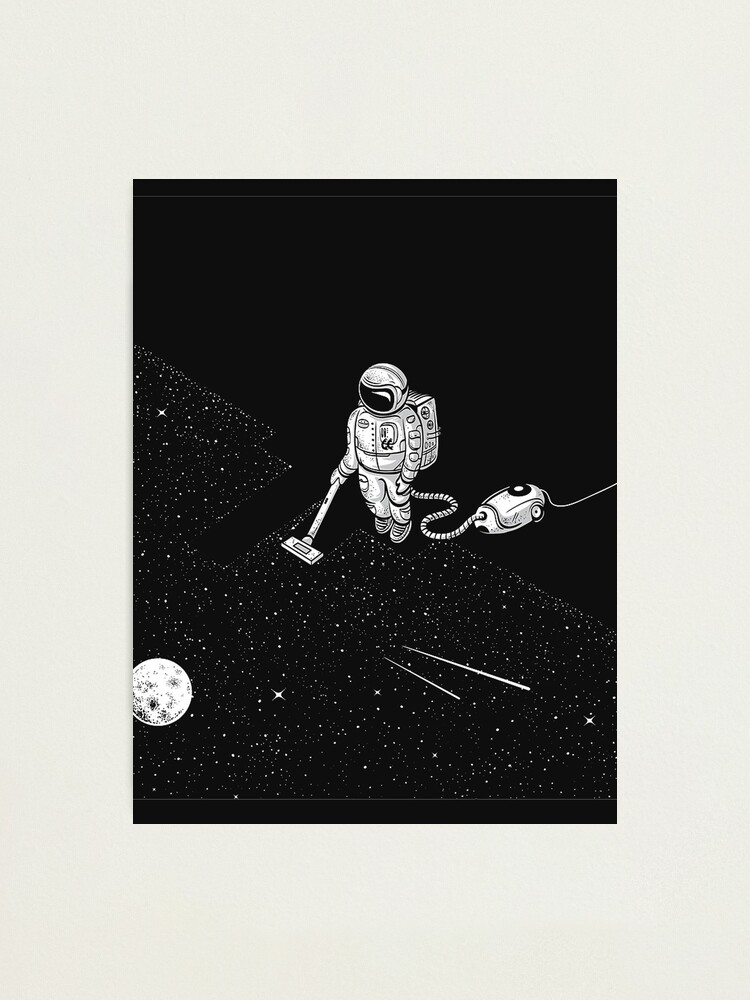The artwork is a vertically-oriented rectangular illustration with a cream-colored background. At the center, there's another rectangle with a velvety black background. This striking piece features an astronaut dressed in a spacesuit, complete with a round helmet and a dark face visor. The astronaut is depicted holding a canister vacuum in their right hand, which has an elongated pipe extending to the front. In a whimsical twist, the astronaut is vacuuming the star-filled night sky.

In the bottom left of the image, a glowing moon or planet is visible. Scattered throughout the sky are dazzling stars, created with dots and little X shapes featuring luminescent centers, alongside a couple of comet-like shooting stars. These stars and celestial objects form a diagonal line from the top-left to the bottom-right of the image. As the astronaut vacuums, the stars and celestial matter are cleared, leaving a trail of void black space behind. This contrast highlights the surreal and satirical nature of the artwork, as the astronaut appears to be tidying up the universe, rendering the once starry sky into a blank, black expanse.